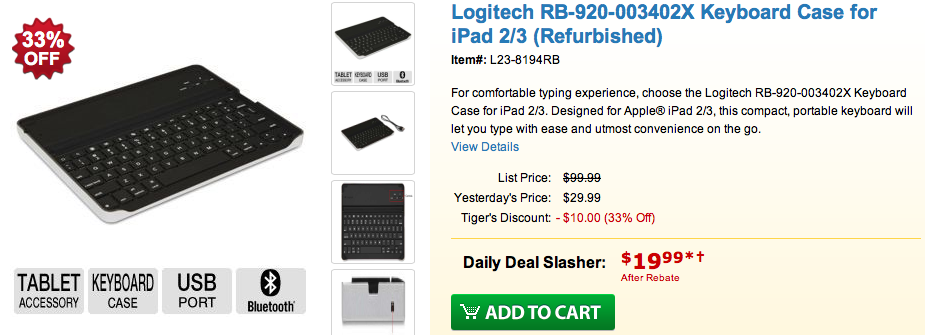This horizontal left-to-right image appears to be a screenshot from a web page or website, accessible via a computer or smart device. The layout comprises a predominantly white background, likely the computer screen's default.

On the left-hand side, there is an image of a black keyboard with a silver rim. A prominent red circle with white text states "33% off". Below the keyboard image, several small gray rectangles feature black text, listing attributes such as "Tablet accessory, keyboard case, USB port, Bluetooth". Additionally, vertically aligned images showcase various details and accessories related to the item.

On the right-hand side, the text "Logitech RB92003402X Keyboard Case for iPad 2/3 Refurbished" is displayed in blue, along with the item number. A brief description follows, and there's a clickable blue "View Details" link. The pricing information is detailed, with the original list price crossed off, followed by "Yesterday's Price: $29.99". The text indicates "Tiger's Discount: -$10, 33% off", with a long yellow line separating this section. Below, "Daily Deal: $19.99 plus" is written in black, accompanied by a green "Add to Cart" button.